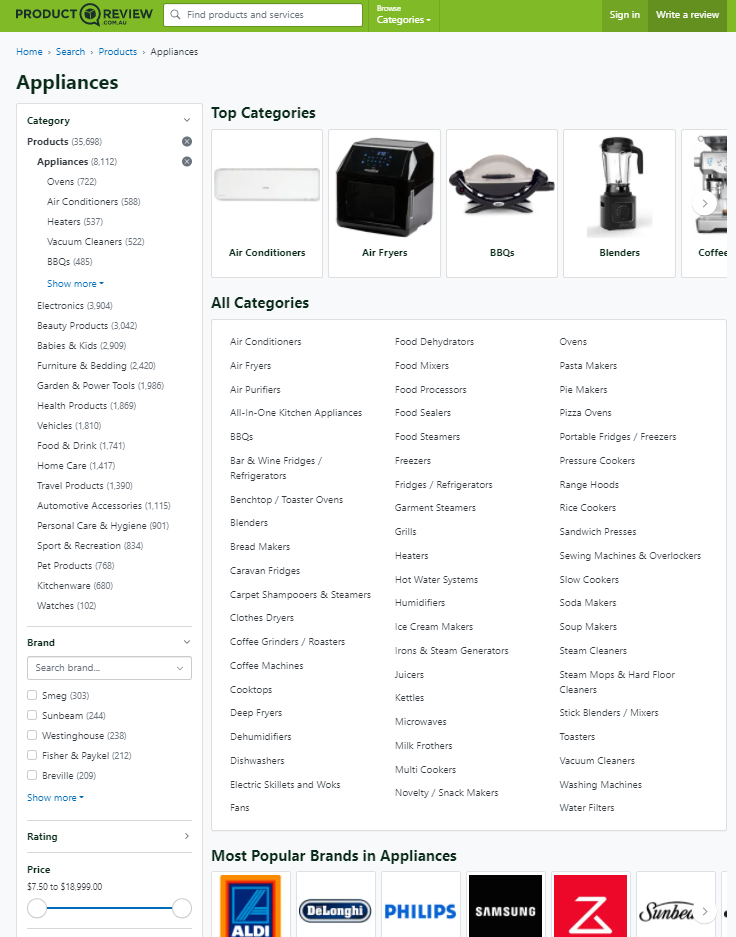The screenshot features a detailed interface of a product review website, characterized by a green header prominently displaying options such as "Sign In," "Write a Review," and navigation categories including "Appliances." Beneath this header, the page organizes content into a list format, housing elements such as product brands, user ratings, and pricing details. A dynamic pricing bar allows users to set minimum and maximum price ranges using two adjustable circles.

Additionally, the site categorizes products under two comprehensive sections: "Top Categories" and "All Categories." "Top Categories" includes items like air conditioners, air fryers, barbecues, blenders, with the category for coffee makers partially cut off. The "All Categories" expands to cover barbecues, air fryers, cooktops, deep fryers, fans, and juicers. 

At the very bottom of the page, it highlights "Most Popular Brands in Appliances," listing brands such as Aldi, Philips, Samsung, and Sunbeam.